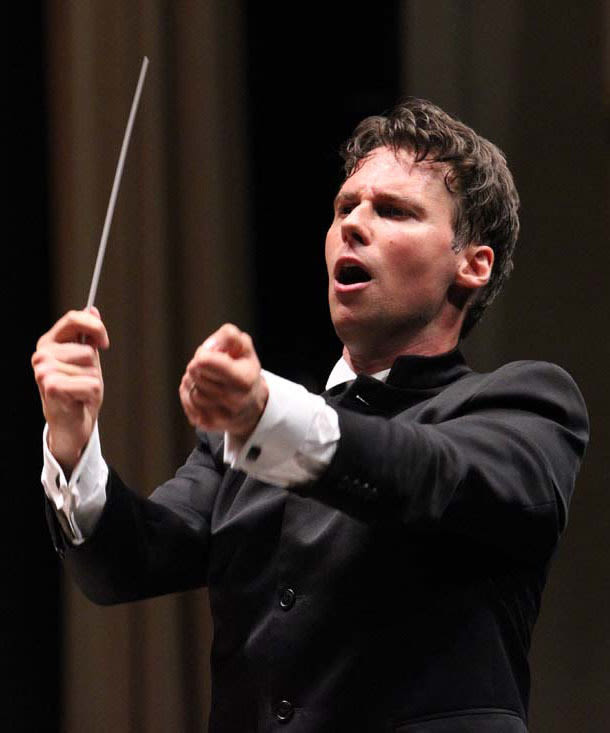The photograph captures a Caucasian male orchestra conductor, appearing to be in his mid-30s to early 40s, with short brown hair that is slightly graying at the sideburns. He is wearing a meticulously buttoned black tuxedo jacket paired with a white collared, long-sleeved shirt, the French cuffs of which are adorned with large black square cufflinks. His black jacket features unique large buttons extending from his neck to his waist, with the top button left undone. As he stands with a serious, furrowed brow expression and his mouth open, potentially mid-command or singing, he holds a small conductor's baton in his right hand, grasping it firmly with his thumb and index finger, and the baton is pointed towards the top left of the image. He is visibly exerting himself, with slight perspiration on his face, which is a bit red. His left hand, lifted in conducting stance as well, displays a wedding band. The background consists of dark-colored curtains, possibly off-white and dark brown, enhancing the dramatic atmosphere of the scene.